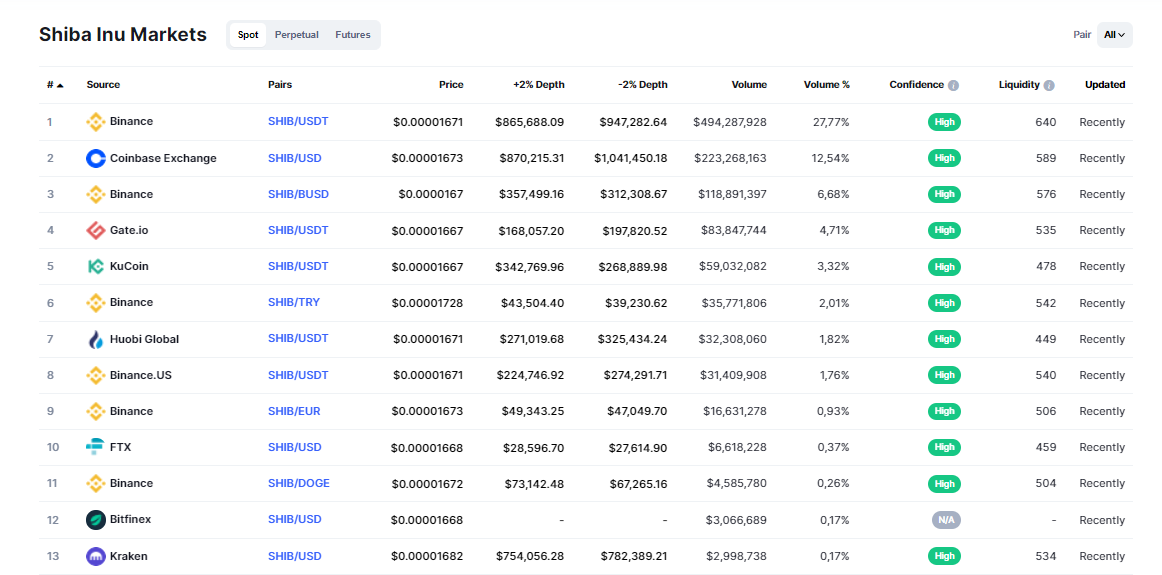**Detailed Screenshot Caption:**

The screenshot displays a segment from the "Shiba Inu Market" interface, set against a white backdrop. In the upper left corner, in black font, the text reads "Shiba Inu Market". Adjacent to this, within a small gray rectangle, the words "Spot Perpetual Futures" are noted, with "Spot" clickable beside it.

Directly beneath, a list spans from item 1 to 13, each encapsulated within white rectangles. Item number 1 at the top showcases the platform "Binance". Associated with Binance, the details are as follows:
- Trading pair: "SHIB/USDT"
- Current price: "$0.0000001671"
- 24-hour trading volume: "$865,688.09"
- 24-hour price change: "$947,282.64"
- Market capitalization: "$494,287,928"
- Price change in percentage: "27.77%"
- A red button indicator labeled "high" in white font
- Additional data: "640 recently"

This detailed list continues in a similar format, enumerating different financial metrics for various companies from positions 2 through 13.